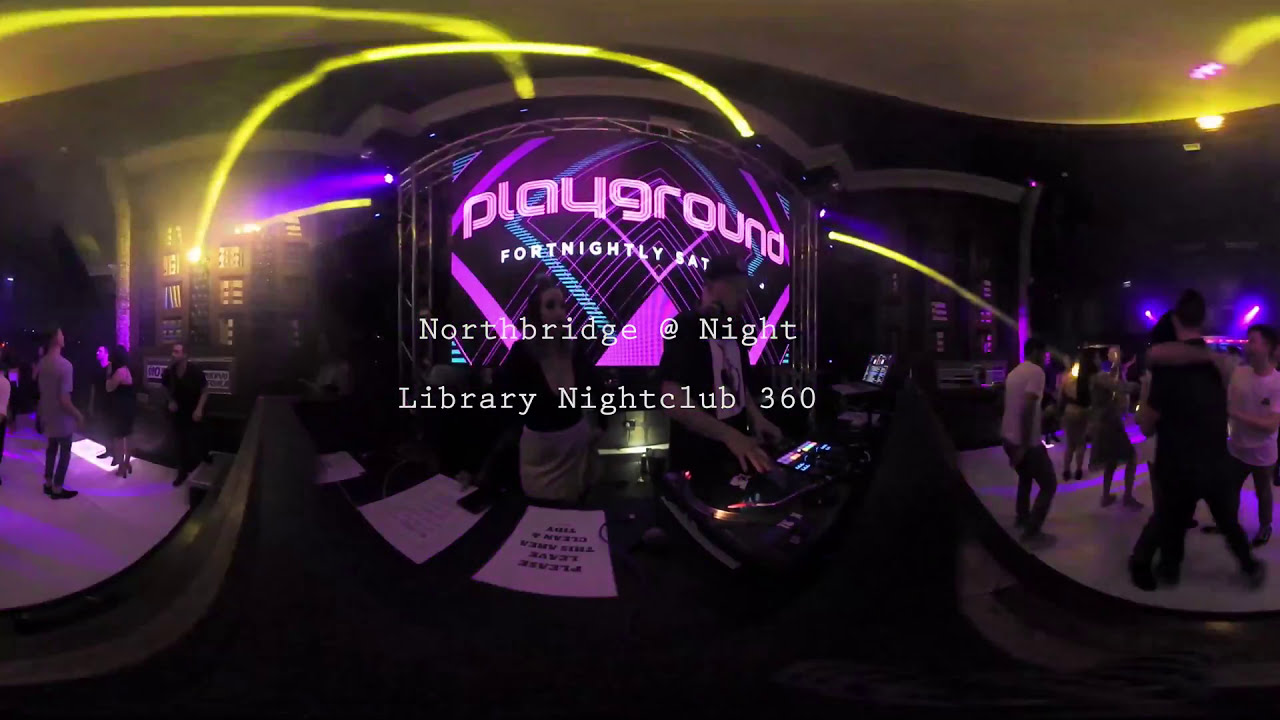The image is a composite, panoramic-like photograph of an indoor nightclub dubbed "Library Nightclub 360," rendered with a fisheye effect. Illuminated by a mix of purple and yellow lights, the nightclub features a white ceiling and contrasting black background walls. Central to the image is a DJ booth framed by a digital display that reads "PLAYGROUND," with additional text displaying "Fortnightly Saturday" and a superimposed "North Bridge at Night, Library Nightclub 360" in white script. Two DJs preside over turntables: a lady dressed in a tan skirt and black shirt, accompanied by a paper with indecipherable black writing in front of her, and a man in a black shirt and hat. On either side of the booth are white dance floors illuminated by vibrant purple lights. On the left, dancers mostly clad in dark clothing, except for one in a white shirt and grey pants, mingle and move energetically. To the right, more dancers, including individuals in black and white attire, amplify the lively atmosphere under the kaleidoscopic lighting. Random yellow arcs of light decorate the ceiling, adding to the vivid and bustling nightclub scene.